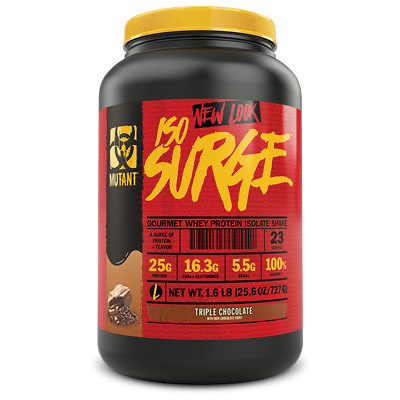This image features a large, black plastic container with a yellow cap, resembling a protein powder jar. It is set against a pure white or transparent background, likely indicating that it is an online store product photograph. The container possesses a prominent red label, which has various inscriptions and details. At the top of the label, within a black banner, the words "New Look" are displayed in red letters. Large yellow stylized font is used for the product name, "ISO Surge," drawing significant attention. Below the product name, in black text, it states "Gourmet Whey Protein Isolate." Further down in yellow text, nutritional information and additional stats are provided, including the weight, "1.6 pounds." Towards the lower end of the label, a brown banner features the words "Triple Chocolate" in white lettering, accompanied by an image of a piece of chocolate on the left side, indicating the flavor of the protein powder.